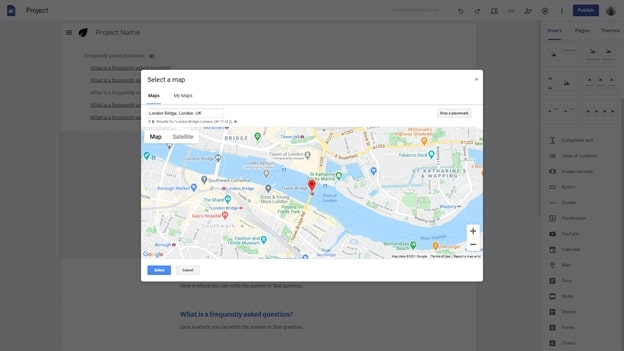This image captures a screenshot of a webpage featuring a user interface for a map-based project. The background of the page is a light black color. 

In the top left corner, there's a dark, slightly out-of-focus square or rectangle with a small indiscernible white image inside. To its immediate right, the word "Project" is prominently displayed in black letters. Adjacent to this, moving right, the header includes a series of icons: a search bar, forward and backward navigation buttons, a profile button, and, on the far right, a publish button. The profile button appears again, repeating at the farthest right of the screen.

Below this header, in the background, the top left corner features a menu button, next to which there is an image of a leaf and the text "Project Name." Below this, there is a dropdown menu with six categories, although these are too blurry to read clearly.

On the right side of the screen, there is another series of menus that are slightly out of focus. These include layout buttons arranged in two by two formations with three rows, and below these, several other buttons that are too blurred to identify.

Dominating the foreground, at the center of the webpage, is a large map with a white background. At the top left of this section, the text "Select a map" is prominently displayed in bold black letters. Towards the far right of this section is a black "X" button. Underneath the "Select a map" text, the menu is highlighted with "Maps" on the left and an out-of-focus word following "Fully" to the right.

Further down, there is a search bar with the placeholder text "London Bridge, London, UK." Below the search bar, a horizontal rectangle displays a selection option with "Map" in bold black letters on the left and "Satellite" in gray letters on the right. At the bottom of this section, a light blue button, likely labeled "Publish," is noted, and next to it on the right is a white button with black letters that possibly say "Layout."